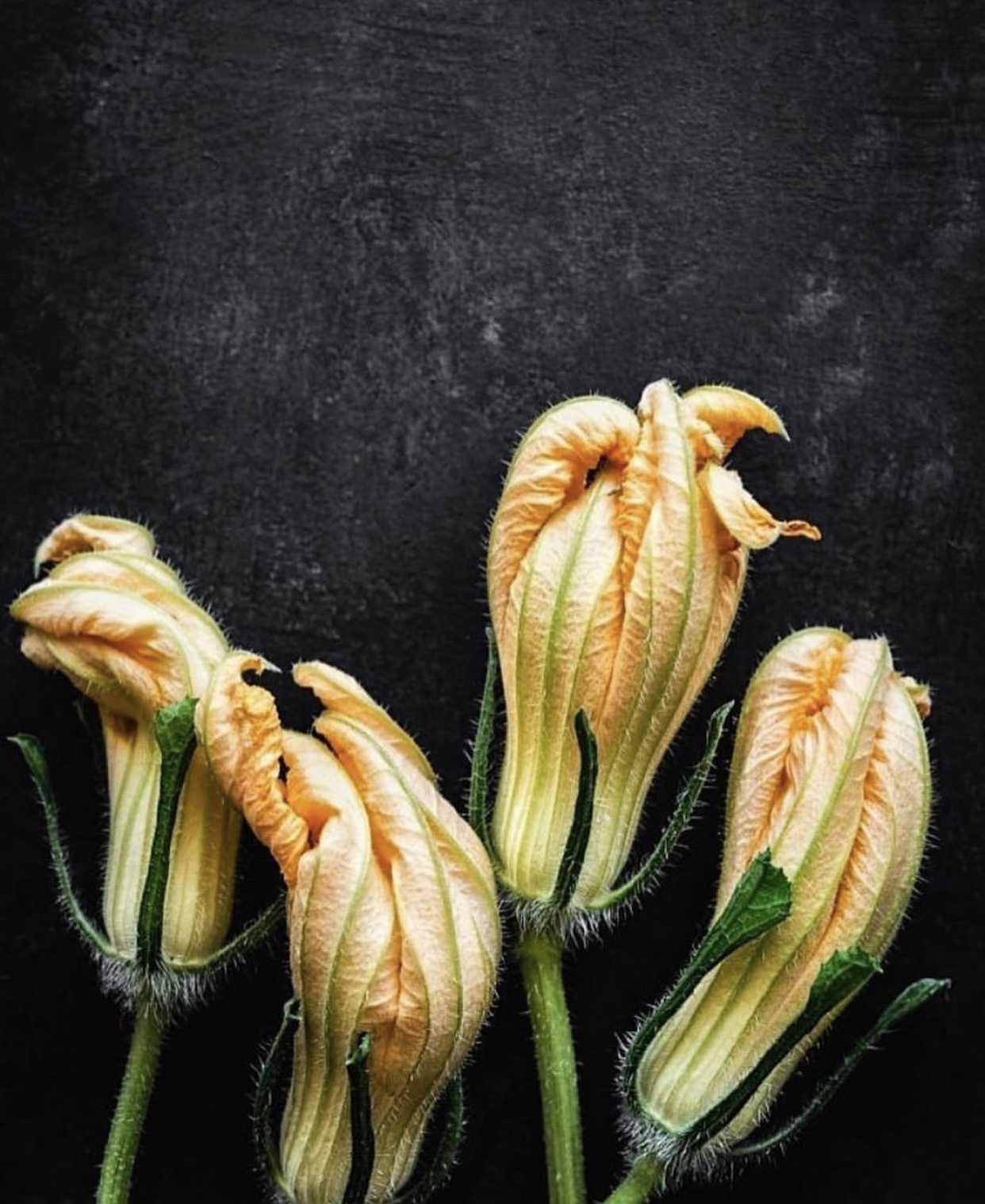The image is a close-up photograph of four wilted, unopened flower buds positioned mostly below the center of the frame. The background is a dark charcoal or faded black wall, possibly with some white or fluff-like markings. From left to right, the first flower has a visible green stem coming up from the bottom left, surrounded by green, fluffy leaves. The bud is light tan or yellow in color, with a slightly prickly texture resembling the inside of a romaine lettuce head. The second flower shows only its peachy-yellow, cantaloupe-colored bud, with green stems in front of it. The third flower, in the best focus and slightly above the others, also features a green pod with white, furry elements at its base. Its stem is visible too. The final flower has a stem that angles sharply to the right before curving back left, leading to another unopened yellow pod surrounded by prickly green stems. The floral arrangement appears to be overlapping, giving a slightly wilted impression.